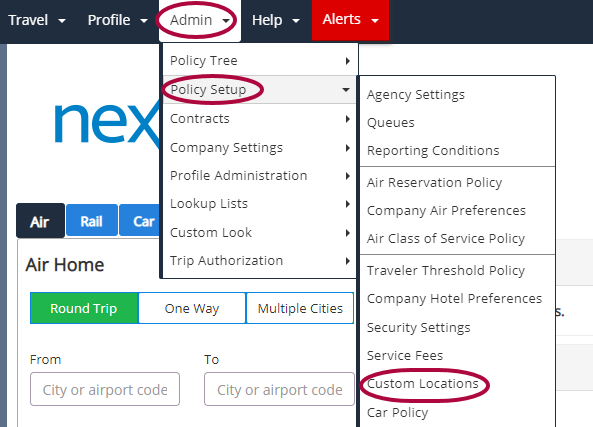The image depicts a detailed view of a search page with multiple dropdown menus and interface options tailored for travel management. At the top of the interface, there are three primary menu options labeled "Travel," "Profile," and "Admin," each accompanied by a dropdown arrow for further selections. The "Admin" dropdown menu is actively expanded, revealing a comprehensive list of administrative functions: "Policy Tree," "Policy Setup," "Context," "Company Settings," "Profile Administration," "Backup Lists," "Custom Look," "Trip Authorization." Among these, the "Policy Setup" dropdown is further opened, displaying several sub-options including "Agency Settings," "Queues," "Reporting Conditions," "Air Reservation Policy," "Company Air Preferences," "Air Class of Service Policy," "Traveler Threshold Policy," "Company Hotel Preferences," "Security Settings," "Service Fees," "Custom Locations," and "Car Policy."

Highlighted in red circles are the words "Admin," "Policy Setup," and "Custom Locations," likely indicating their importance or selection. In the background of the interface, additional elements are visible, such as the word "NEX" as well as categories like "Air," "Roll," "Rail Car," "Air Home," "Road Trip," "One Way," and "Multiple Cities," providing a comprehensive tool for managing travel arrangements and policies. The overall layout is complex and detailed, indicating robust functionality for travel management and administration.